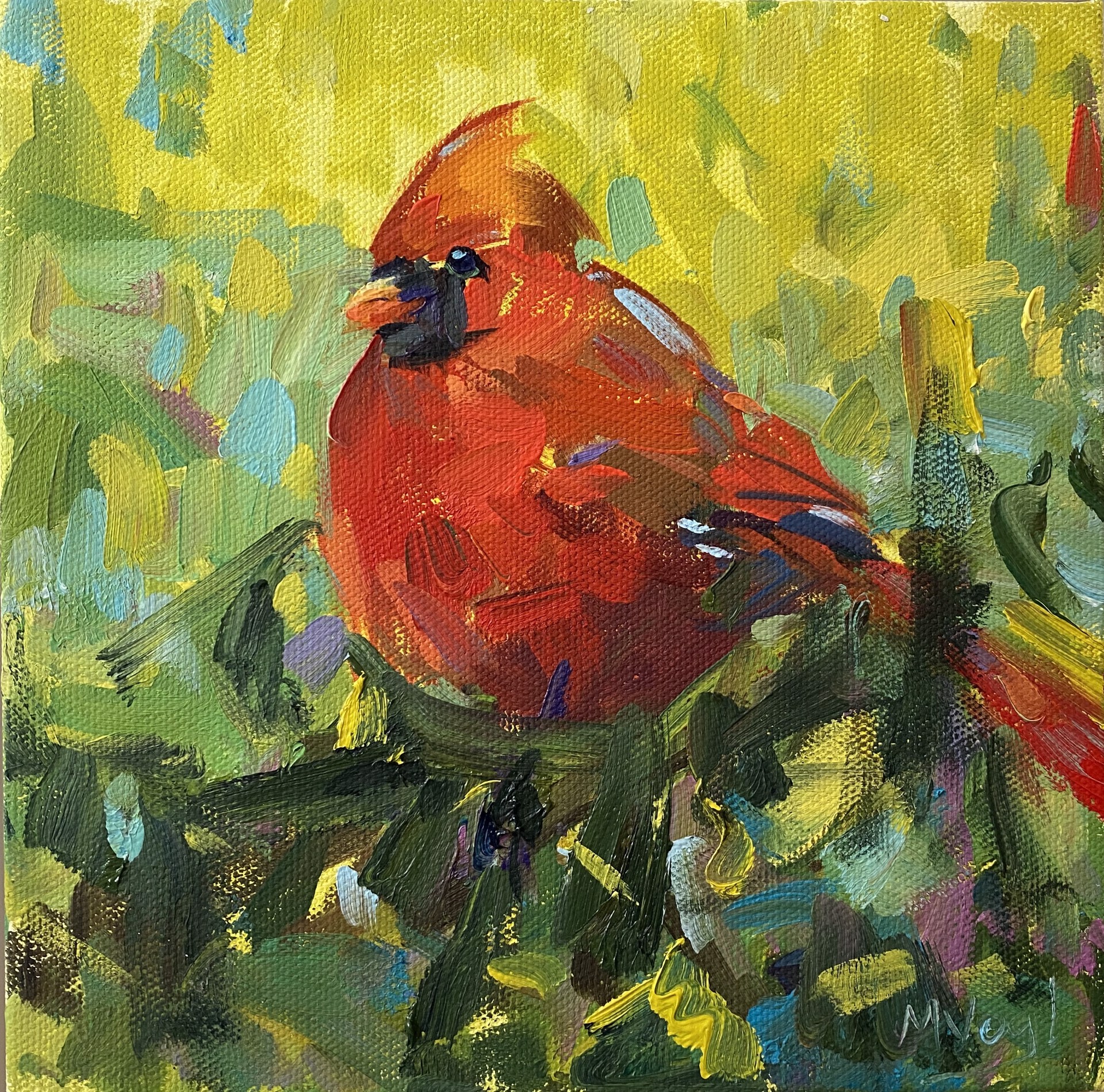This painting portrays a plump red bird, possibly a cardinal or red-breasted robin, characterized by an orange rounded beak surrounded by black feathers and a striking black, beady eye. The bird's vibrant red body features hints of blue and yellow streaks, as well as accents of white and black feathers, adding to its detailed and striking appearance. The painting is highly stylized and abstract, with rough, unblended brush strokes in various directions that create an impressionistic background of greens, yellows, blues, reds, and purples. This background likely represents elements of nature such as trees, grass, flowers, and sky, but remains vague and undefined. The bird seems to be perched, although it's unclear whether it's on a branch or nestled in the grass due to the painting's abstract nature. A signature in the bottom right corner, difficult to decipher but possibly reading M-V-E-G-L or M-Y-A-G-L, marks the artist's identity.